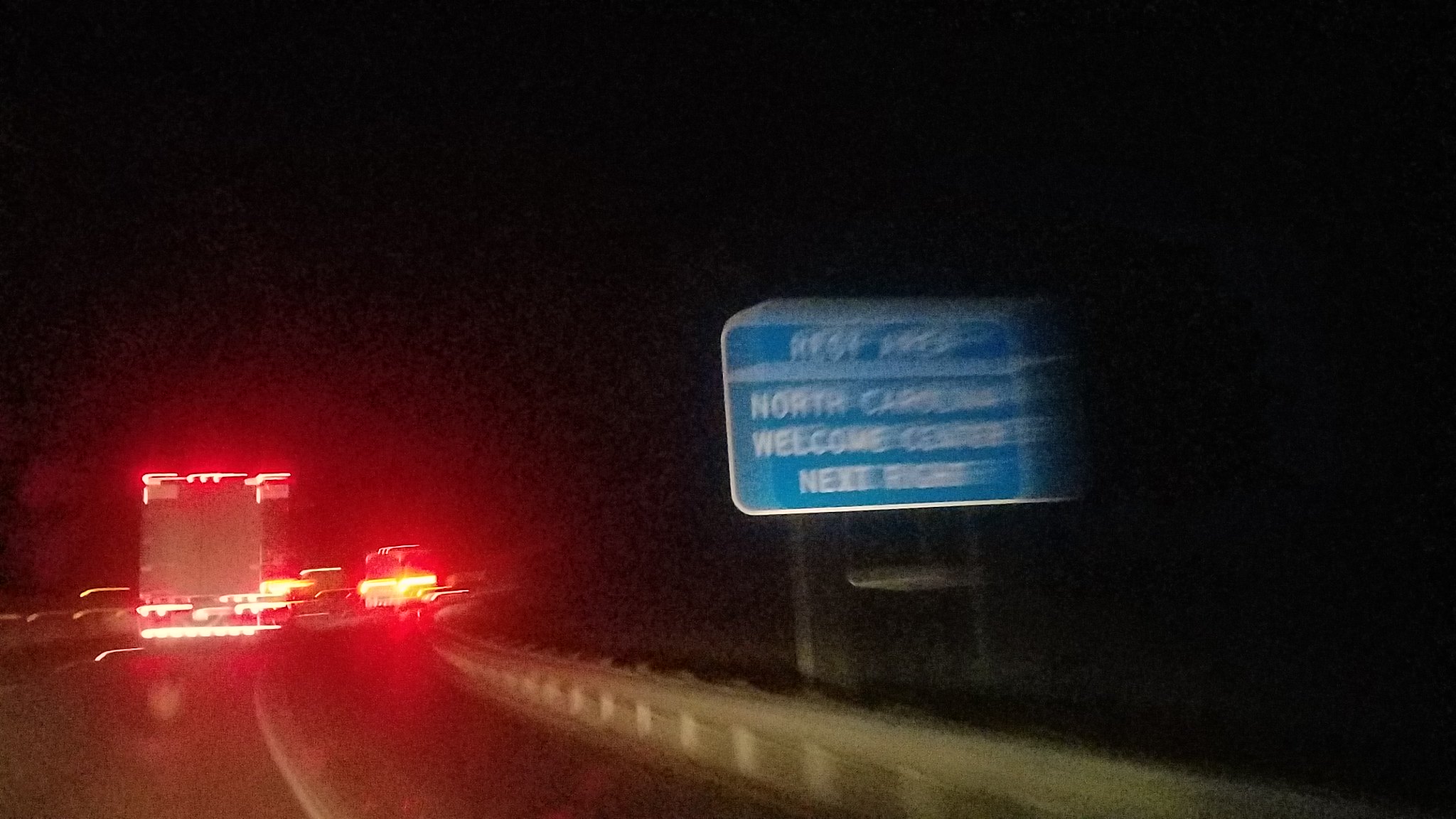A captivating nighttime photograph portrays a car driving down a highway, with a semi-tractor trailer and other vehicles visible ahead, their taillights creating a vibrant red glow in the distance. On the right side of the road, a gray guardrail runs parallel to the white lane marking. A roadside sign, though slightly blurred due to motion, can be discerned rising on two gray posts. The sign, bordered in white with a sky-blue background, appears to read: "Rest Stop North Carolina Welcome Center Next Right", adding a touch of clarity amid the evening's haze.